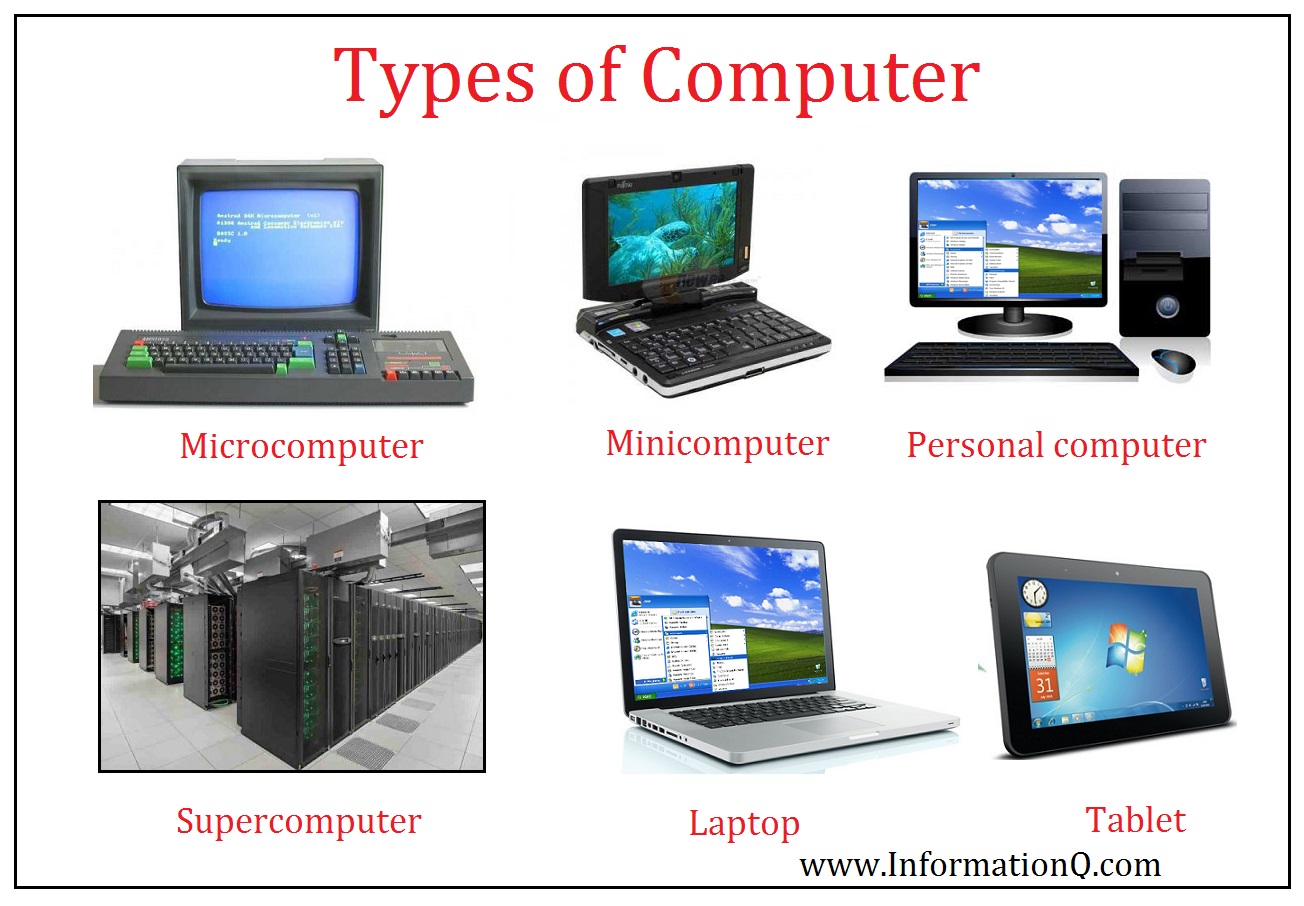The image showcases various types of computers against a white background with a black border. At the top center, the heading "Types of Computer" is displayed in red text. Below the heading are two rows of images, each depicting a different type of computer with labels beneath them in red text. 

In the top row, from left to right, are: 
- A microcomputer with a blue screen and thick keyboard,
- A minicomputer featuring an underwater screensaver,
- A personal computer displaying a sky background with multiple windows open.

In the bottom row, from left to right, are: 
- A supercomputer taking up an entire room,
- A laptop,
- A tablet showcasing the Windows icon.

In the bottom right corner, still within the border, the text "www.informationq.com" is displayed in black letters. The diverse appearances and forms of each computer type are vividly illustrated, providing clear visual distinctions among them.